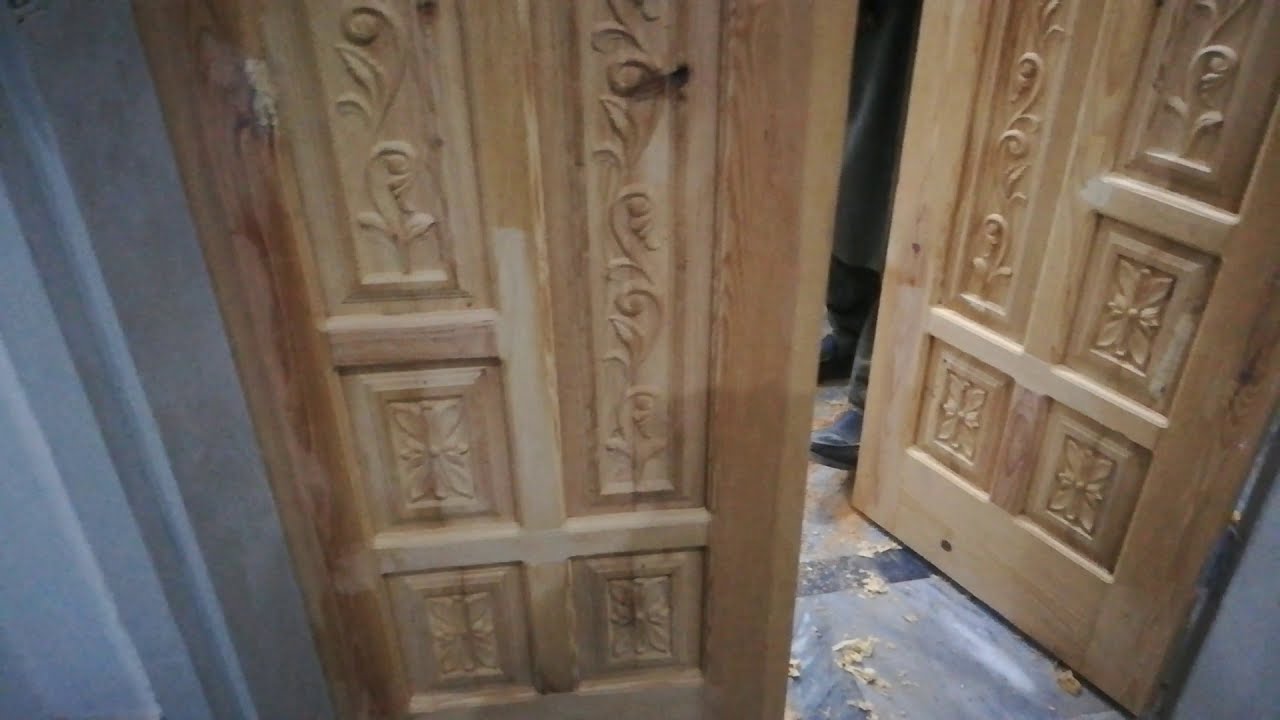The photograph or photorealistic image depicts an ornate double doorway made of light-colored, unfinished wood, featuring intricate carvings of swirls, vines, and flowers on each panel. Both identical doors meet in the middle, but the right door is slightly opened, revealing a glimpse of the room beyond. The floor inside is a gray stone, speckled with lighter chips. The image, shot from above, captures the legs of a person partially obscured by the door and the top edge of the image. The person is wearing brown shoes, brown pants, and a long black coat. The doorway is flanked by white walls with a stony appearance.